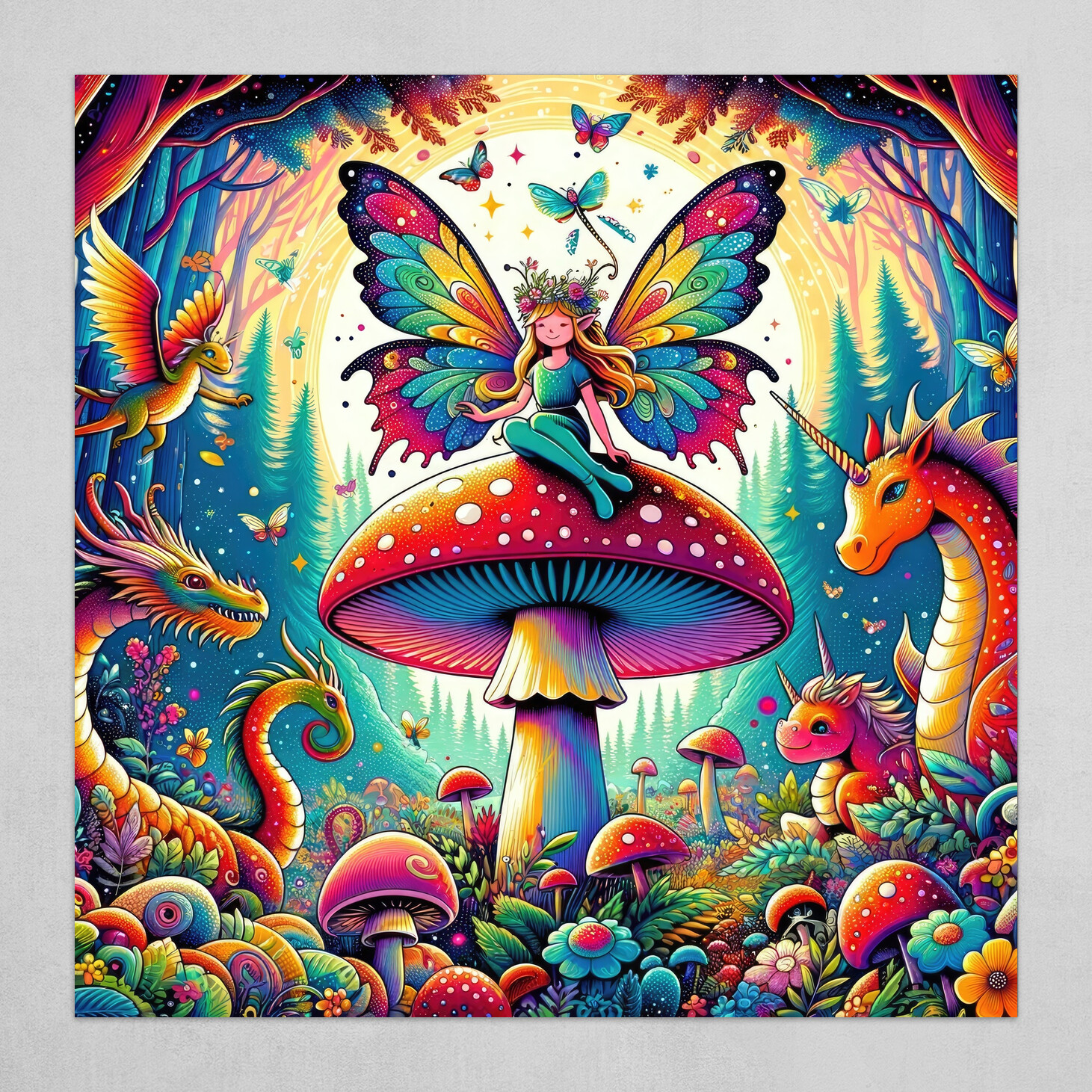This vivid, fantasy scene is a detailed, psychedelic drawing, likely created with colored pencils or markers. At its center is a large, multi-colored mushroom with a red cap that fades to orange, yellow, and white, set against a tie-dyed backdrop of rainbow hues. Perched on this mushroom is a female fairy with butterfly wings in a spectrum of colors, adorned with a crown of flowers in her blonde hair, dressed in a blue tunic and leggings. She is enveloped in a fantasy forest teeming with neon branches and a variety of brightly colored mushrooms in shades of pink, purple, yellow, and blue.

Surrounding the fairy are various fantastical creatures: on the right, several unicorns, including one in the foreground and glimpses of others peeking from behind trees; to the left, multiple dragons of different forms—some feathery and long-necked, others more bulky with horns and lizard-like features. Among them, a flying salamander and a small dinosaur add to the mystical ambiance. Butterflies and dragonflies flutter around, accentuating the fairy's luminescence cast by the sun directly behind her, which bathes the scene in radiant light.

The backdrop is a forest landscape with trees in shades of reds, bronzy browns, and blues, enhancing the surreal, otherworldly atmosphere. This intricate tapestry or poster-like artwork exudes a fantastical charm through its brilliant use of vivid colors and imaginative elements, creating a mesmerizing, enchanted forest realm.